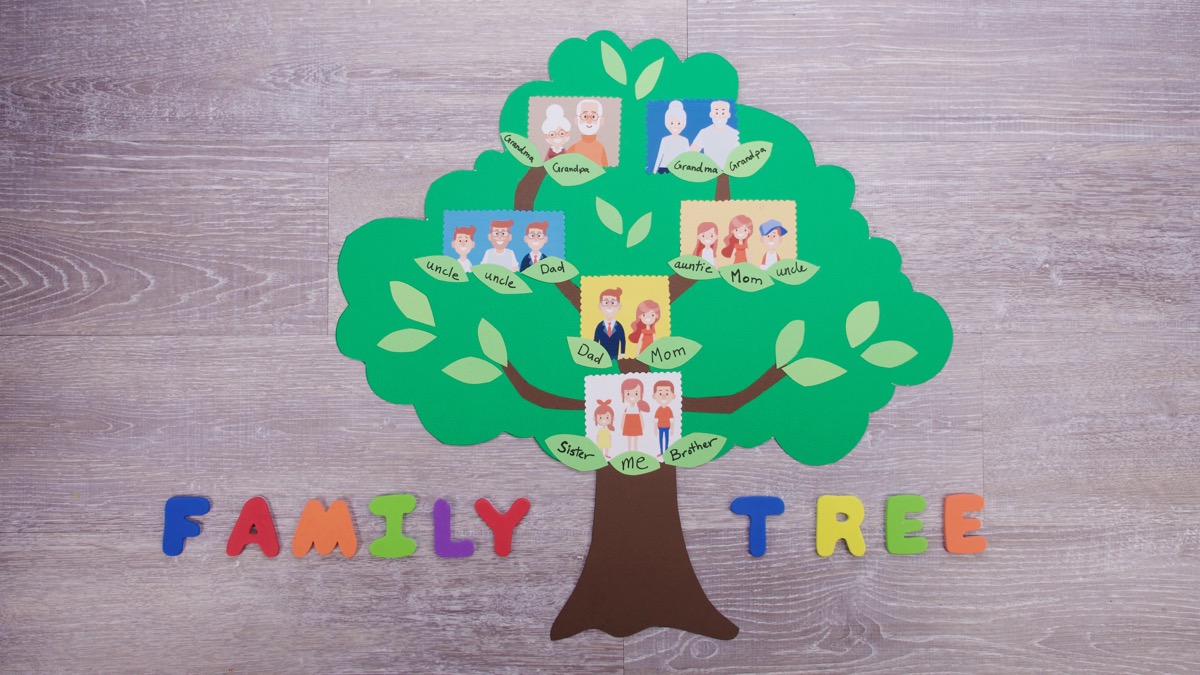This detailed family tree project is a colorful display likely created by a child for a school assignment. The main feature is a construction paper cutout of a tree with a green canopy and brown trunk, arranged either on a wooden paneled wall or a hardwood floor. At the bottom, "Family Tree" is spelled out in bright, primary-colored letters. The tree is adorned with cartoonish photos of family members, organized into a tiered structure. At the very top of the tree are two sets of grandparents, each labeled Grandma and Grandpa. Below them, the branches divide to show two sets of family members: on one side, Uncle, Uncle, Dad, and on the other side, Auntie, Mom, Uncle. Further down are the child's parents, labeled Dad and Mom. Finally, at the base of the tree, closer to the trunk, are the siblings: Sister, Me (a female figure), and Brother. This engaging depiction highlights the child's extended family connections in a vibrant and organized manner.